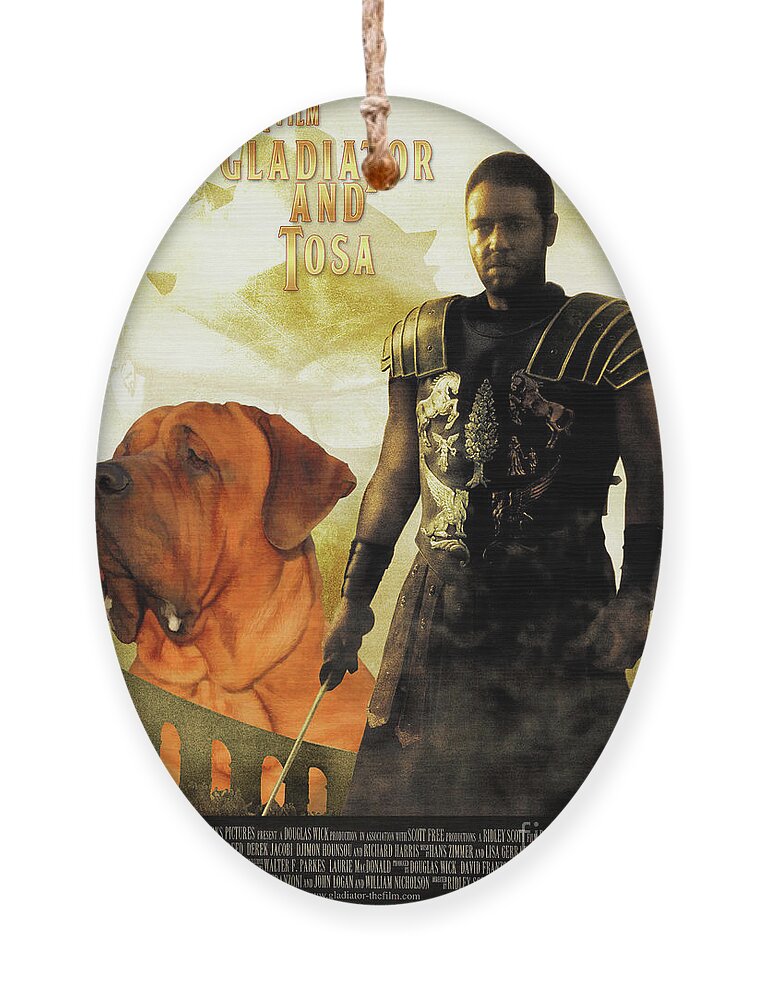The image appears to be a digital edit depicting an oval-shaped medallion or trinket designed to resemble a movie poster. Central to the medallion is a detailed illustration of Russell Crowe's character from the movie "Gladiator," clad in full armor and holding a gladius in his right hand. To his left stands an orange bulldog, seemingly looking towards the left in a three-fourths view. The top of the medallion has the text "Gladiator and Tosa" prominently displayed. There is a hole at the top of the medallion through which a string is threaded, creating the appearance of a necklace. The entire scene is set against a white background with professional studio lighting, highlighting the medallion's intricate details and enhancing the composition.